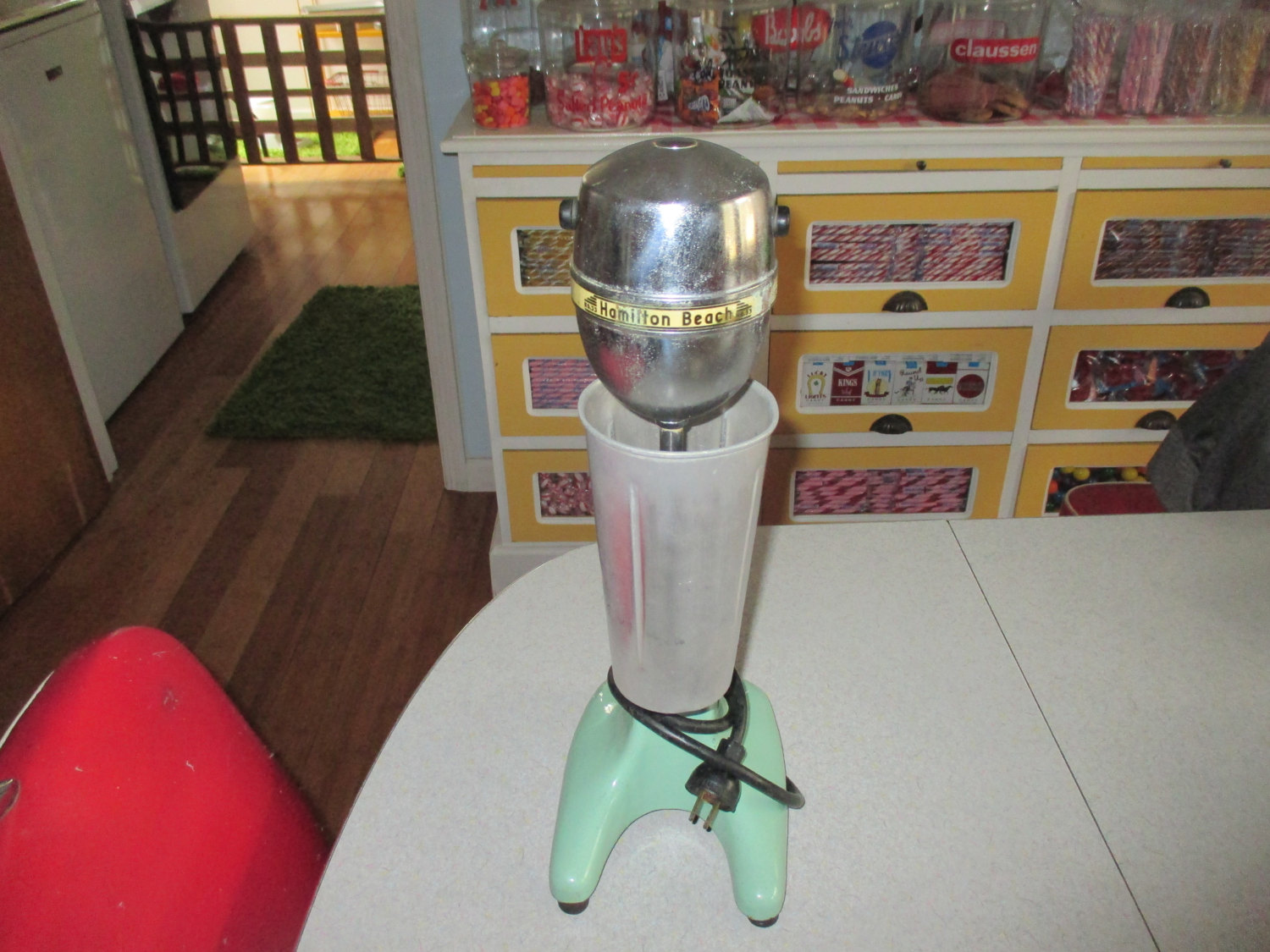The image depicts a vintage Hamilton Beach mixer prominently placed on a white Formica table surrounded by red chairs. The mixer features a light turquoise base with a wrapped power cord and a plastic mixing cup. The metallic top, engraved with "Hamilton Beach," integrates a metal shaft that extends into the cup. In the background, yellow drawers with detailed labels display contents, while the countertop above holds large glass jars filled with various candies, including peppermint and sour balls. The room’s wooden flooring and a small brown carpet are partially visible, along with a netted barrier in the doorway, likely for pet or child safety, lending a nostalgic ambiance to the scene.